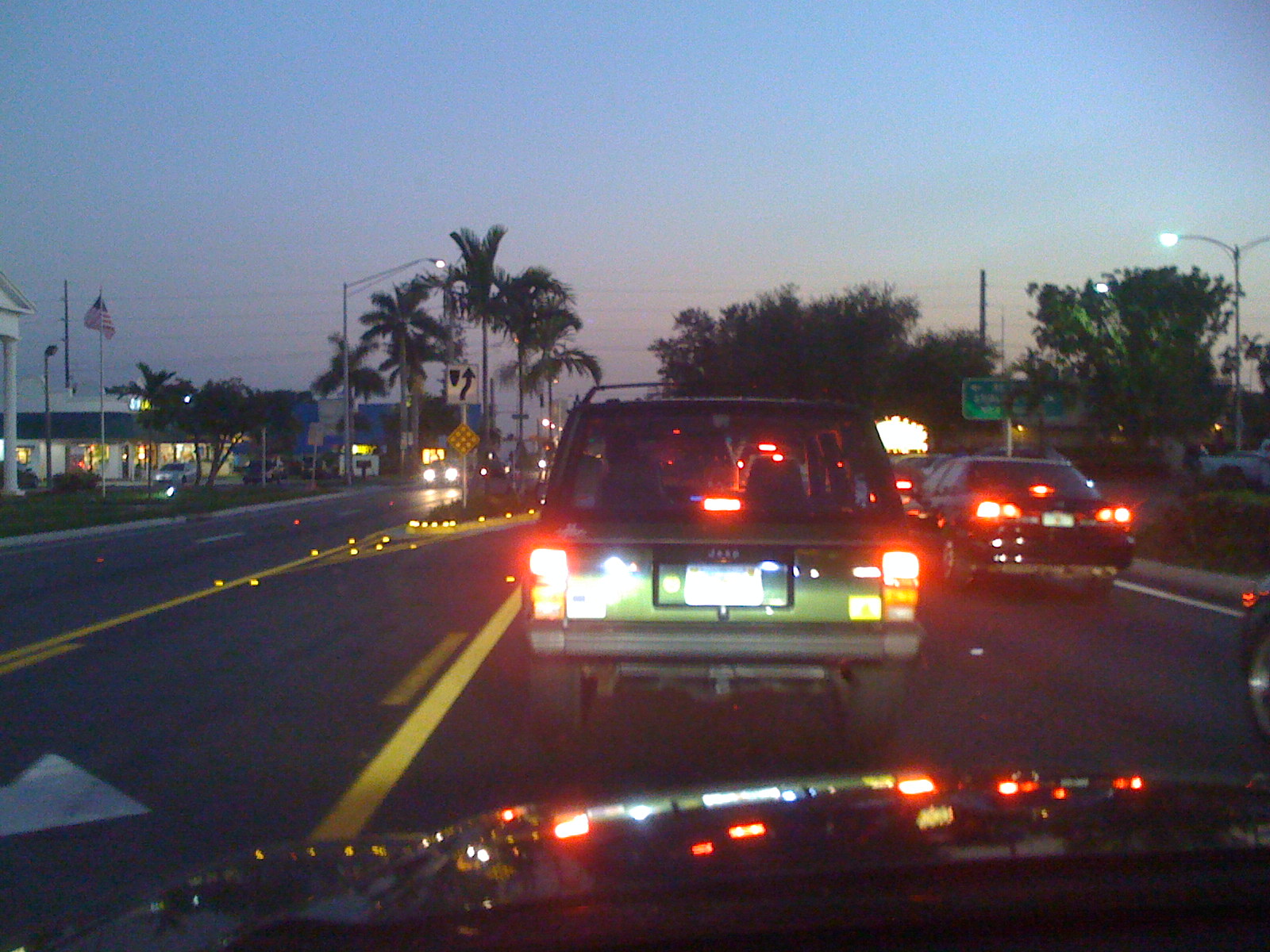The image, taken from inside a car caught in traffic, captures a bustling four-lane highway with a central turn lane, framed by city lights and palm trees. The scene appears to be at dusk, with the sky painted in blue, purple, and pink hues as the sun sets. Directly ahead, a green Jeep SUV has its brake lights illuminated, indicating a stop. The polished, dark-colored hood of the car reflects the myriad of streetlights and vehicle lights around. To the sides of the road, various businesses and gas stations are lit up, including a recognizable McDonald's. An American flag on a white pole stands prominently against the twilight backdrop. Additional details include a white sign with a black arrow and yield sign situated in the median, and several big palm trees lining the center area. Heavy traffic is evident, with numerous cars visible in both directions, their taillights and headlights creating a sea of red and white lights. The streetlights are already on, casting a glow over the scene, and the overall atmosphere is one of a typical busy evening transitioning into night.